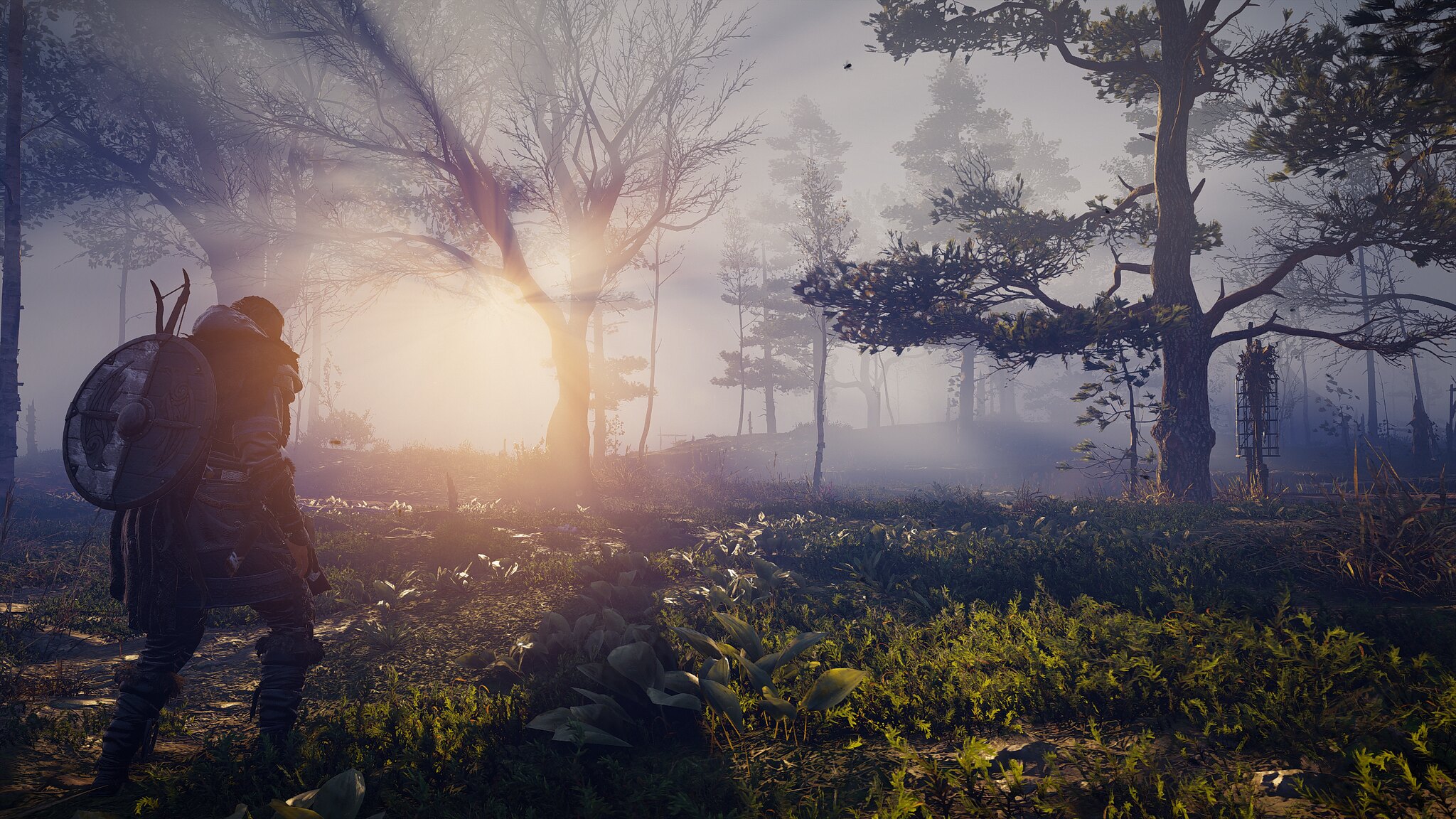The image is a detailed artwork likely depicting a scene resembling Assassin's Creed Valhalla. It features a Viking-era character, seen from behind, who appears to be on a hiking trail at dawn. The character, clad in a fur coat, leather-like outfit, and big boots, carries a distinctive round shield with a blue and white design and a bow and arrow on his back. The scene captures him walking through a dense, foggy forest with a mix of barren and leafy trees, and green plants dotting the grassy pathway. The sunlight is just starting to rise to the top left of the image, casting a soft glow over the landscape and enhancing the serene, yet adventurous ambiance.